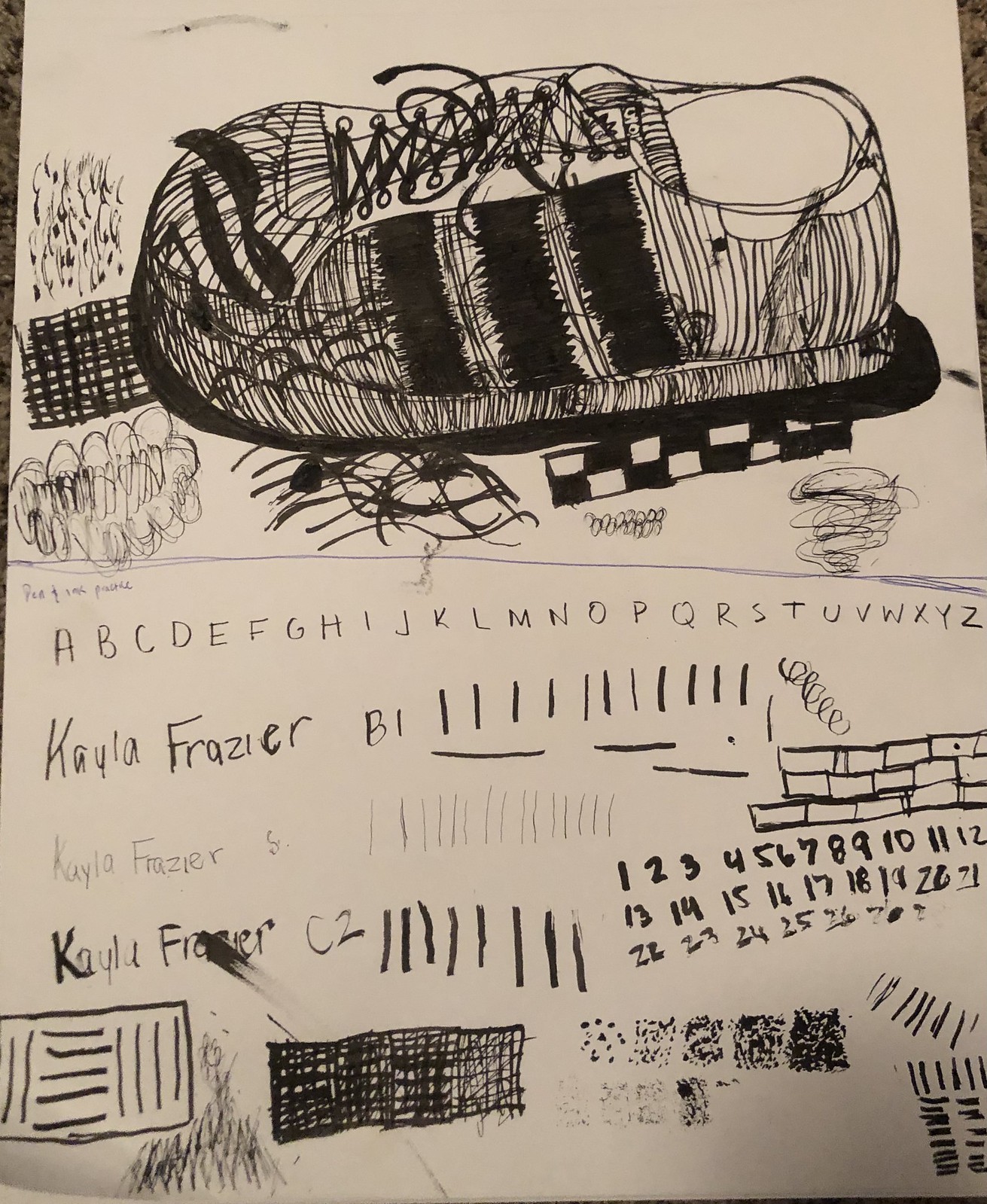On a granite surface, a white page adorned with various doodles and drawings captures attention with its intricate details. Dominating the page is a large, meticulously crosshatched drawing of a shoe, complete with three distinct shadows that enhance its depth and dimensions. The artist has illustrated the shoe's contours and texture with fine precision.

Directly below the shoe, a domino effect pattern and a suede circle pattern add an interesting visual contrast. In front of the shoe, crosshatching and curly lines further enrich the composition. Beneath these elements, the entire alphabet from A to Z is neatly inscribed, showcasing a range of typography experiments.

Prominent among the doodles is the word "Caliphrysia," surrounded by various other whimsical scribbles. The artwork appears to be created by a child exploring different printing and artistic styles, using both fine-tip and thick-tip black pens to bring their imaginative expressions to life. The border of the image prominently features the texture of the granite surface, grounding the playful scene in a tangible reality.